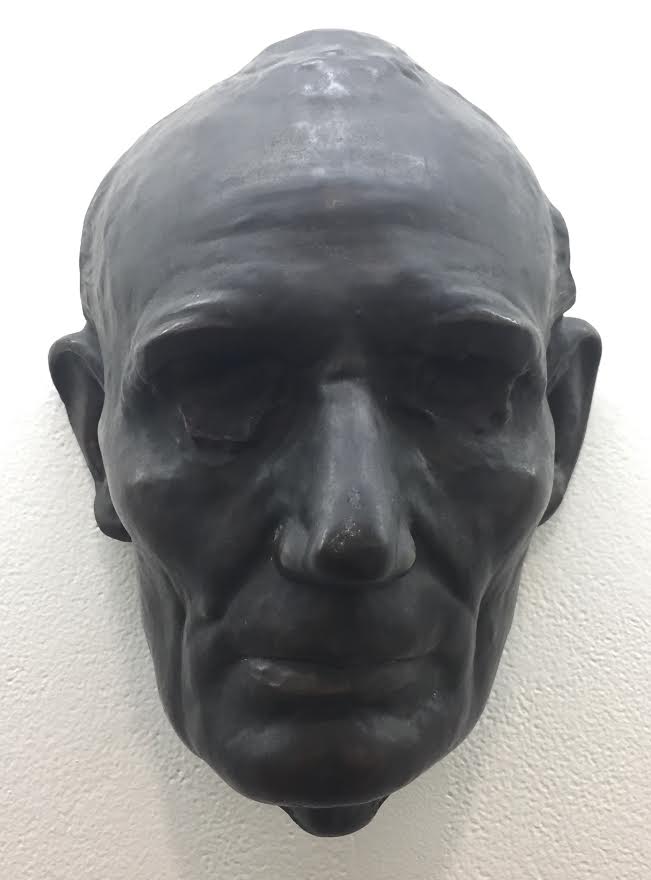This photograph features a detailed marble or stone sculpture of an elderly man's head mounted on a white, possibly stucco, wall. The sculpture, predominantly gray in color, depicts a head with sunken cheeks, a pronounced, somewhat lumpy nose, and significant ears. The hair is sparse, primarily around the sides, leaving the crown and forehead more exposed, which reflects light. The eyes are deep cavities, accentuating the hollow look and adding to the expressionless demeanor of the face with its closed mouth. The forehead bears visible markings or textures, and the chin exhibits some loose skin. The wall behind the head starts as completely white in the upper half and transitions to an off-white towards the bottom of the image, where a slight shadow from the sculpture can be seen. This photograph appears to be taken indoors, capturing the solitary, well-preserved sculpture with minor wear around the nose.